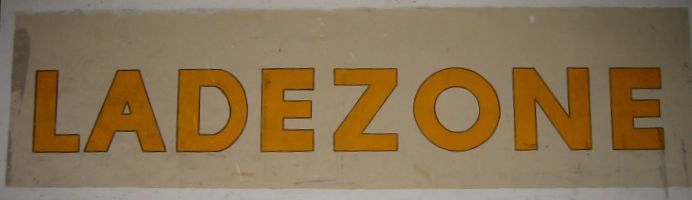This photograph features a stenciled name on a wall. The wall appears to be either white or tan in color, serving as the backdrop for the prominent text. The name "LADE ZONE" is stenciled in bold, block letters, which have been filled in with a vivid orange color. The lettering suggests it was either drawn in with a pen and then colored or spray-painted to achieve its striking finish. The meticulous craftsmanship of the stencil and the vibrant hue of the letters make the name "LADE ZONE" stand out clearly against the neutral background.